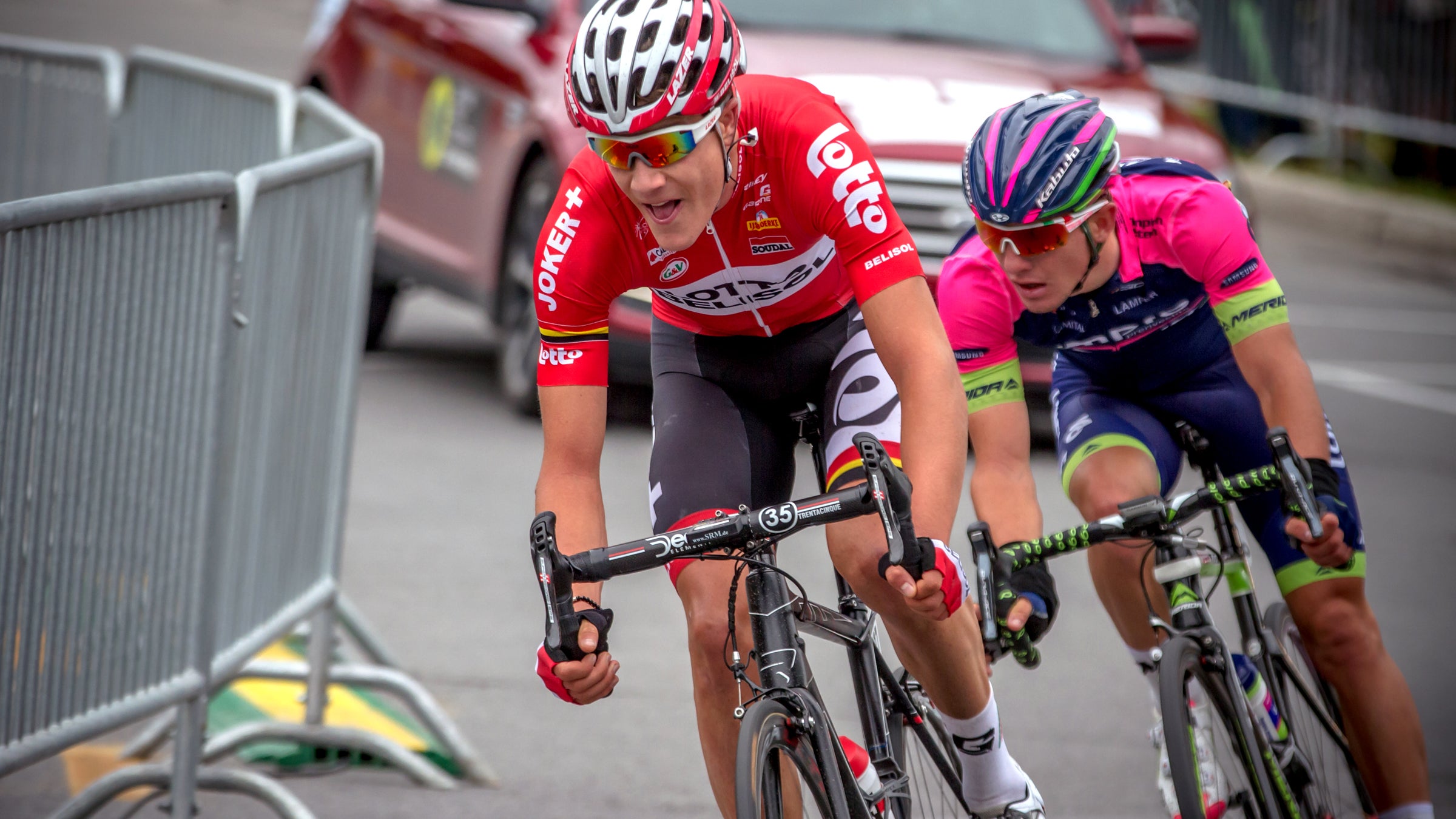This vibrant photo captures two professional cyclists, fully immersed in a race, riding along a fenced-off roadway flanked by caution stripes. The leading cyclist dons a sleek ensemble of tight, black shorts and a vivid red top adorned with white text reading "Joker Plus" and "Lotto Bellasol." He sports a matching red and white helmet marked "LASER" and reflective athletic sunglasses with white rims. Number 35 is visible on the handlebars of his black bike. Trailing slightly behind, the second cyclist wears a striking outfit of blue, pink, and neon green, complemented by a blue helmet with colorful stripes. His black and neon green bicycle stands out as much as his attire. A red escort car, emblazoned with yellow logos, follows closely behind, ensuring the path remains clear for the riders. The surrounding guardrails and the fenced-off area emphasize the competitive setting of the event.